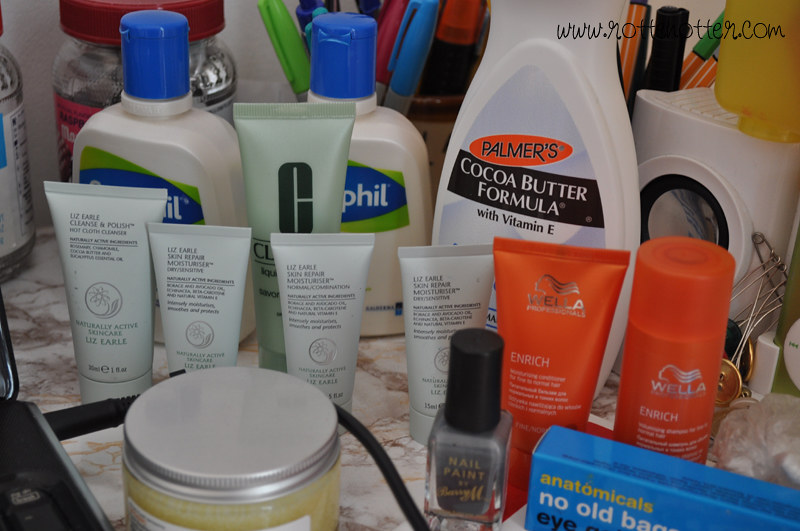This photograph showcases a cluttered bathroom countertop or storage area teeming with a variety of supplies. Prominently in the bottom left-hand corner, a black electronic device is plugged in, with its cable wrapped around a jar featuring an aluminum round top. Adjacent to this, a small bottle of gray nail polish with yellow lettering adds to the assortment. Moving right, a blue box inscribed with yellow, white, and black text reads "anatomicals, no old bag, and I." 

In the following row behind these items, a selection of diverse cosmetic containers is displayed. Among these, there are four containers of varying sizes in light gray and green hues, as well as two vibrant orange containers. Behind them stands an array of skincare products, including a Clinique lotion container, two Cetaphil lotion containers, and a cocoa butter formula by Palmer's. 

The very back of the countertop is lined with cups brimming with assorted Sharpies and other pens, emphasizing the multifunctional nature of the space. To the right, a peculiar item resembling a tiny plastic washing machine can be spotted, along with an assortment of buttons and safety pins, adding to the eclectic mix of items on this busy countertop.